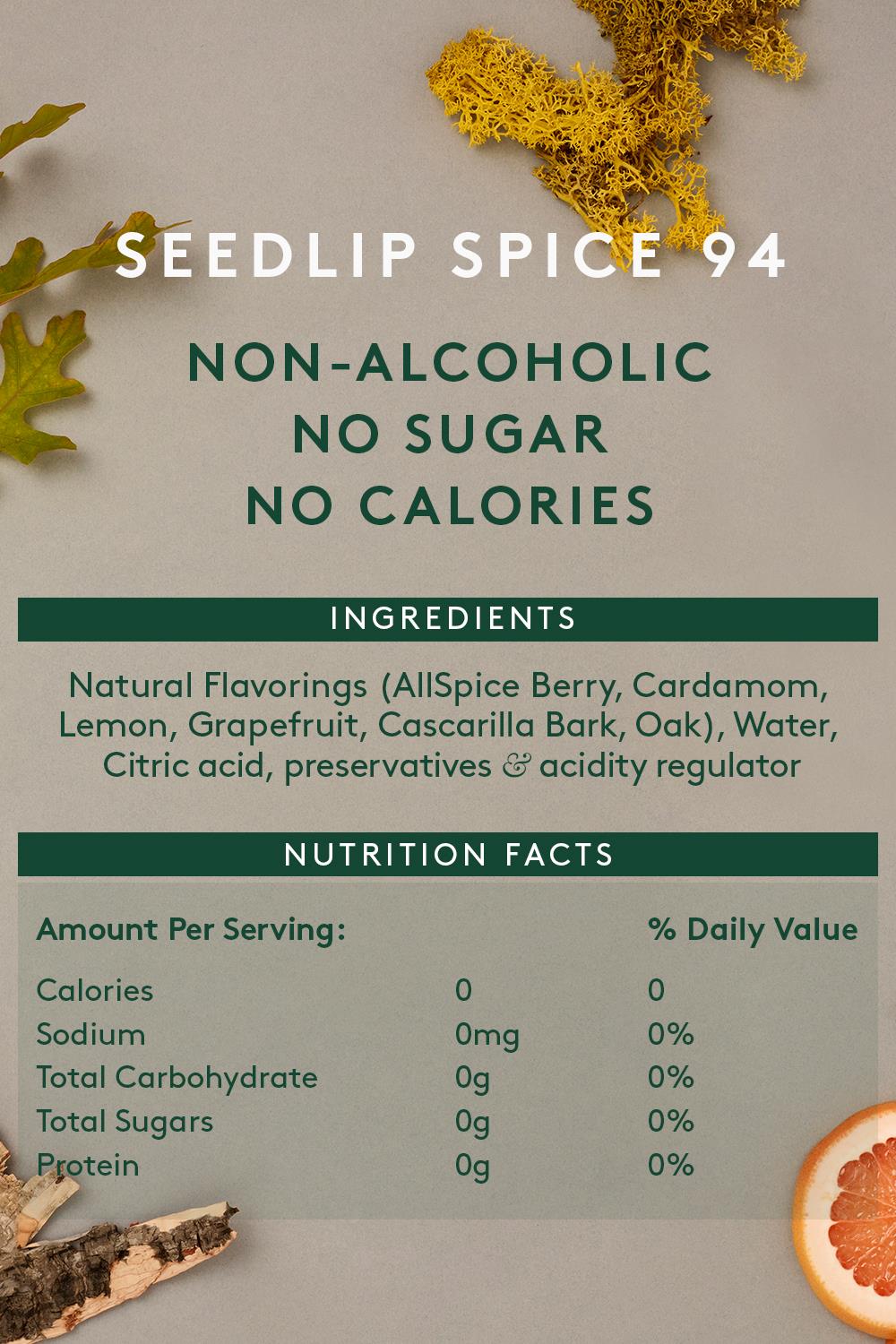The image appears to be a detailed ingredient list for a beverage labeled "Seedlip Spice 94." The text is presented in white and green, with the product name "Seedlip Spice 94" prominently displayed in white text. Beneath it, green text states that the drink is non-alcoholic, contains no sugar, and has zero calories. 

A green bar with white lettering introduces the "Ingredients" section, listing components such as natural flavorings, allspice, berries, cardamom, lemon, grapefruit, water, bark, oak, citric acid, preservatives, and acidity regulators. 

Below this is another green bar labeled "Nutrition Facts" in white letters. This section details various nutritional values, including calories, sodium, carbohydrates, sugars, and protein, all of which are listed as zero, along with their percentage daily values.

The background is a beige-grey color, adorned with various images that provide a visual context for the ingredients. On the bottom right is an image of a half-cut grapefruit, while the upper left features a stick or twig, possibly representing bark. The top left corner shows a leaf, and the top right displays a patch of yellow moss. These elements emphasize the natural ingredients within the beverage.